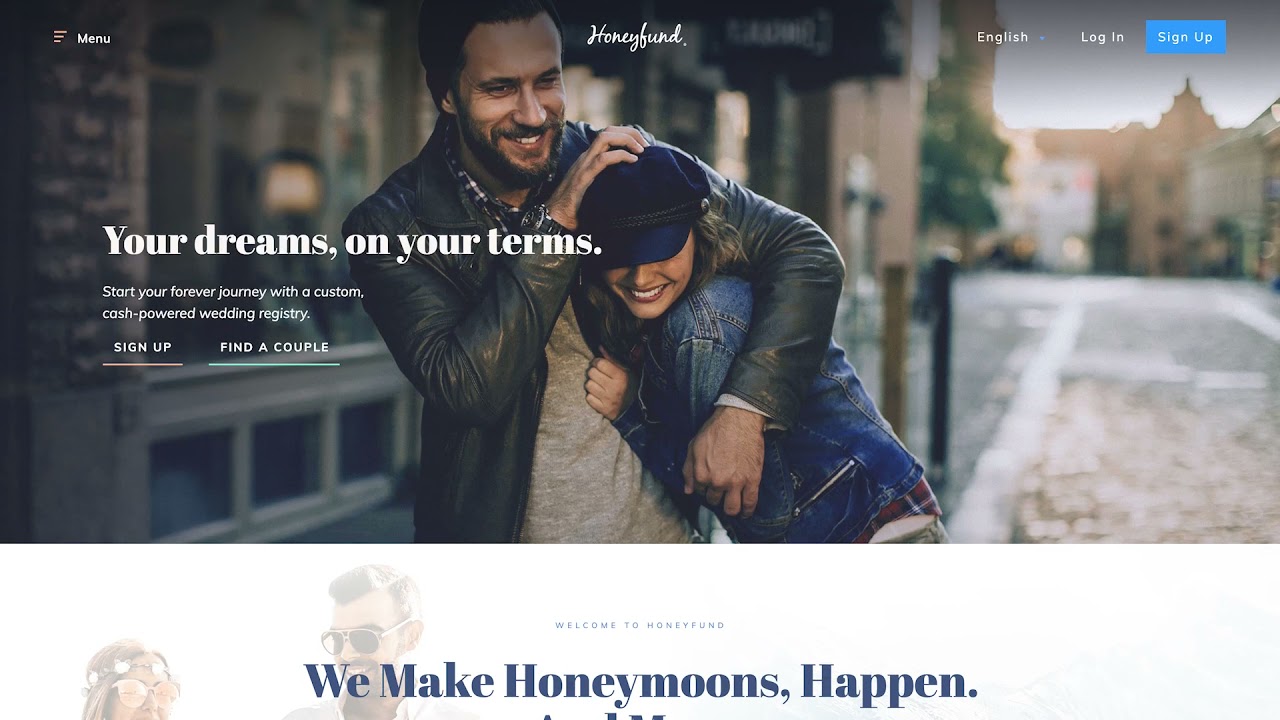This image is a screenshot of a website designed for honeymoons. The layout features a wide horizontal image of a joyful couple strolling down a cobblestone street in a picturesque European neighborhood. The man on the left has a brown beard and wears a reddish beanie, a black leather jacket over a gray shirt, and has his arm wrapped around his partner. She is beaming with a smile, adorned in a blue cap and a blue jean jacket.

As they walk, the sun sets behind them, casting a golden hour glow over the scene and giving the distant European architecture a warm, dreamy quality. The focus of the image is on the couple, with the background elements artistically blurred to accentuate this.

In the top left corner of the image, there's a menu icon alongside the text "Honey Fund" in cursive. The top right corner features options for "English," "Login," and a blue "Sign Up" button. Overlaid on the main image, bold white text reads, "Your dreams on your terms," followed by a smaller font that says, "Start your forever journey with a custom cash-powered wedding registry."

Below this text, there are two interactive options: "Sign Up" and "Find a Couple." At the very bottom of the image, a welcoming message states "Welcome to Honey Fund," accompanied by a prominent blue text declaration, "We make honeymoons happen."